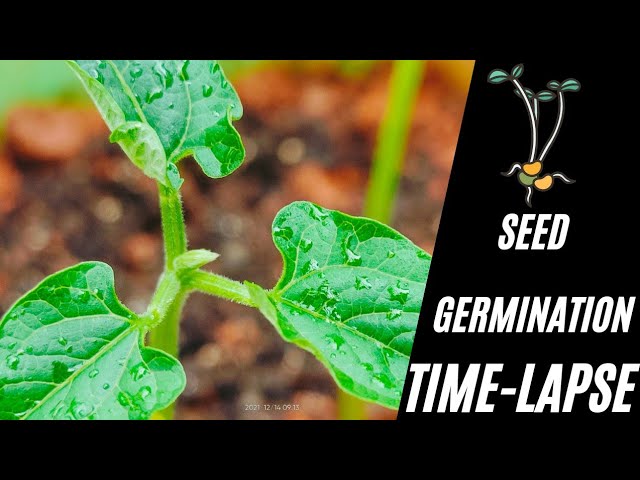The image portrays a small, young plant with three green leaves bearing multiple water droplets, situated against a background of soil that is slightly blurry and reddish-black with a hint of green at the top. This realistic photo is positioned on the left side of the horizontal image, while the right side features an illustrated depiction of a green and yellow plant with narrow stalks and leaves at the top. The right side also includes white text reading "Seed Germination Time Lapse." The image is framed by wide black bands at the top and bottom, and it is marked with the year 2021 at the bottom.